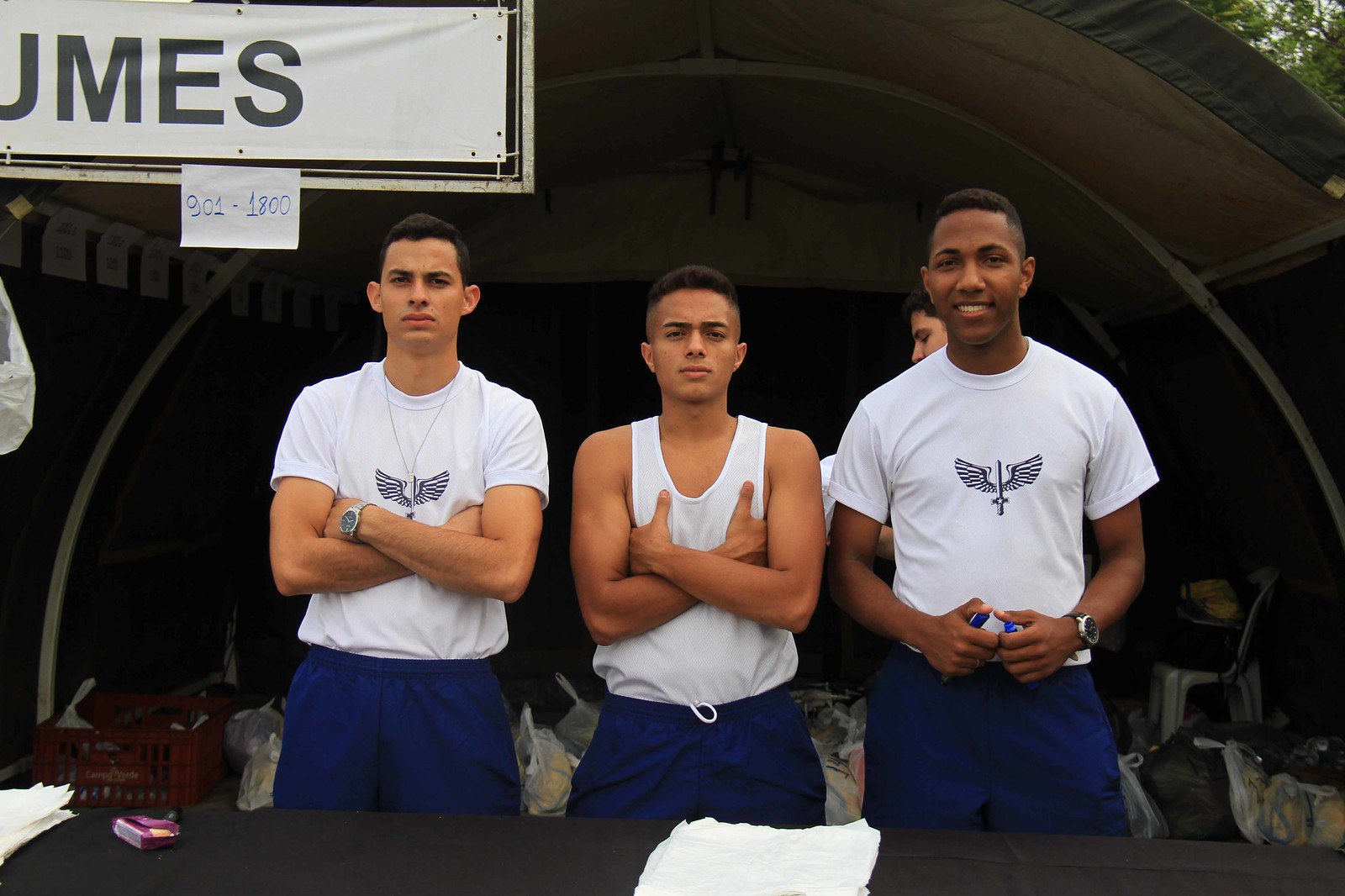In this full-color photograph taken outdoors during the day, three dark-haired young men are posing and staring at the camera, standing in front of an archway or large tent. The white banner in the upper left-hand corner, trimmed in black and gray, displays the partial letters "U, M, E, S" in black font. A piece of regular paper with blue writing showing the numbers "901-1800" is tacked onto the bottom of the banner.

In the foreground, a gray table draped with a towel and possibly holding a pack of cigarettes sits in front of the young men. The three males are dressed in blue pants with white shirts, with the individuals on the left and right donning white t-shirts featuring a sword flanked by eagle wings. The young man on the left wears a watch and has his arms crossed, while the one in the middle, wearing a white tank top or "wife beater," poses with his hands tucked into his armpits, flexing his muscles. The young man on the right is also wearing a watch and the same sword-and-wings adorned shirt as the one on the left. 

Two of the young men, who appear to be Latino with beige-ish green skin tone, are on the left, while the slightly darker-skinned individual stands on the right. The background reveals various bags and equipment cluttered inside the tent-like structure behind them. Additionally, another boy can be seen walking in the background, adding to the lively scene.